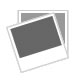The image features a red short-sleeved t-shirt hanging on a white foam-like hanger with a silver hook, set against an entirely white background. The t-shirt displays bold white text at the top spelling out "BROWN" in a curved format. Below this, there is a white rectangular area with red text spelling "ATHLETICS" in all capitals. The hanger is visible but does not appear to be attached to anything, enhancing the clean, minimalist presentation of the t-shirt.